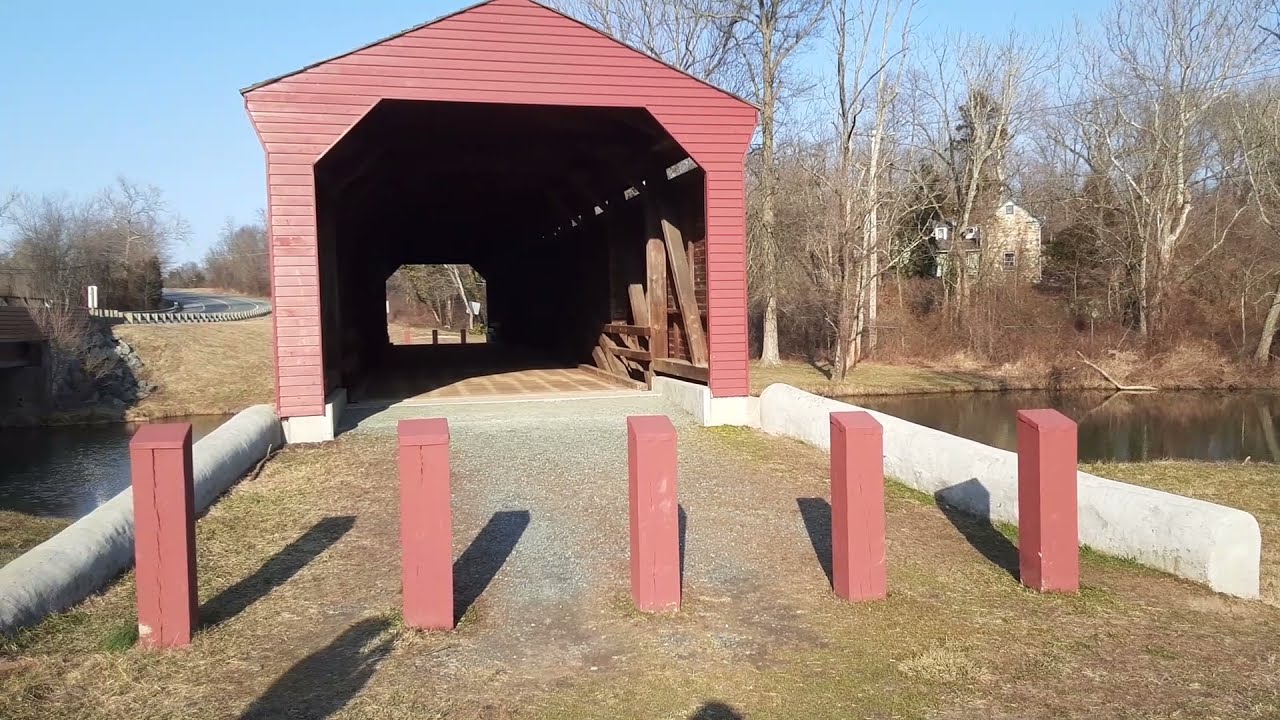The photograph features a prominent red-covered wooden bridge spanning a river that flows from the left to the right of the image. The bridge, which has a triangular roof, is centrally positioned in the frame and creates a dramatic contrast with its surroundings. At the entrance to the bridge, five vertical red poles act as barriers. The river is filled with water and shows parts of a shoreline adorned with dry trees and plants on the right side. Near this shore, a house is visible, adding an element of habitation to the scene. To the left of the bridge, a road stretches into the background, creating a sense of depth. The surrounding area includes various colors like brown, gray, red, tan, blue, white, and yellow, enriched by the blue sky above, indicating the photograph was taken during the day. The exterior of the covered bridge casts a shadow within, creating a dark interior that contrasts with the brightly lit environment outside. Power lines are visible at the top right, further enhancing the detailed outdoor setting. The image is devoid of any text, focusing solely on the natural and man-made elements within the scene.